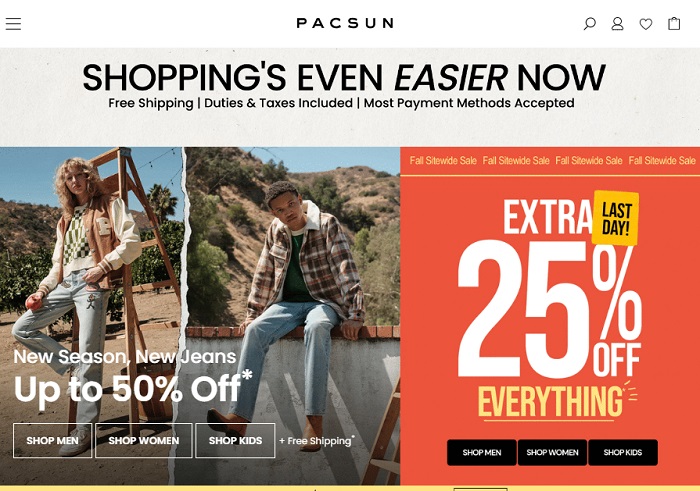This is a detailed description of the Paxson shopping website homepage. At the very top, centered in bold letters, is the brand name "Paxson." To the left of the name, there's a collapsible menu icon, and on the right, a series of icons for search, account, favorites, and cart.

The main section of the page features a prominent banner with the headline, "Shopping is even easier now. Free shipping, duties and taxes included. Most payment methods accepted." This message is displayed in large black letters, making it the focal point of the page.

Below this, there's a vibrant promotional poster. It showcases two individuals styled chicly against an earthy, natural backdrop with a few trees visible.

The first individual is posing confidently in front of a wooden ladder. They are dressed in white-washed jeans, a cardigan, and topped with a baseball jacket. The scenery behind them is muddy and woodland-like.

To the side, the second individual is seated on a brick wall, sporting an ensemble of brown boots, blue jeans, a greenish t-shirt, and an overlapping shirt. 

Overlaying this image is a text that reads, "New season, new jeans, up to 50% off," alongside three call-to-action buttons labeled "Shop men," "Shop women," and "Shop kids," emphasizing the added benefit of free shipping.

Adjacent to the main poster is a smaller, vibrant orange banner offering an "Extra 25% off everything." This banner also includes three similar call-to-action buttons: "Shop men," "Shop women," and "Shop kids."

Altogether, the homepage is designed to immediately draw attention to current promotions and sales, encouraging shoppers to explore various categories with the enticing offers prominently displayed.